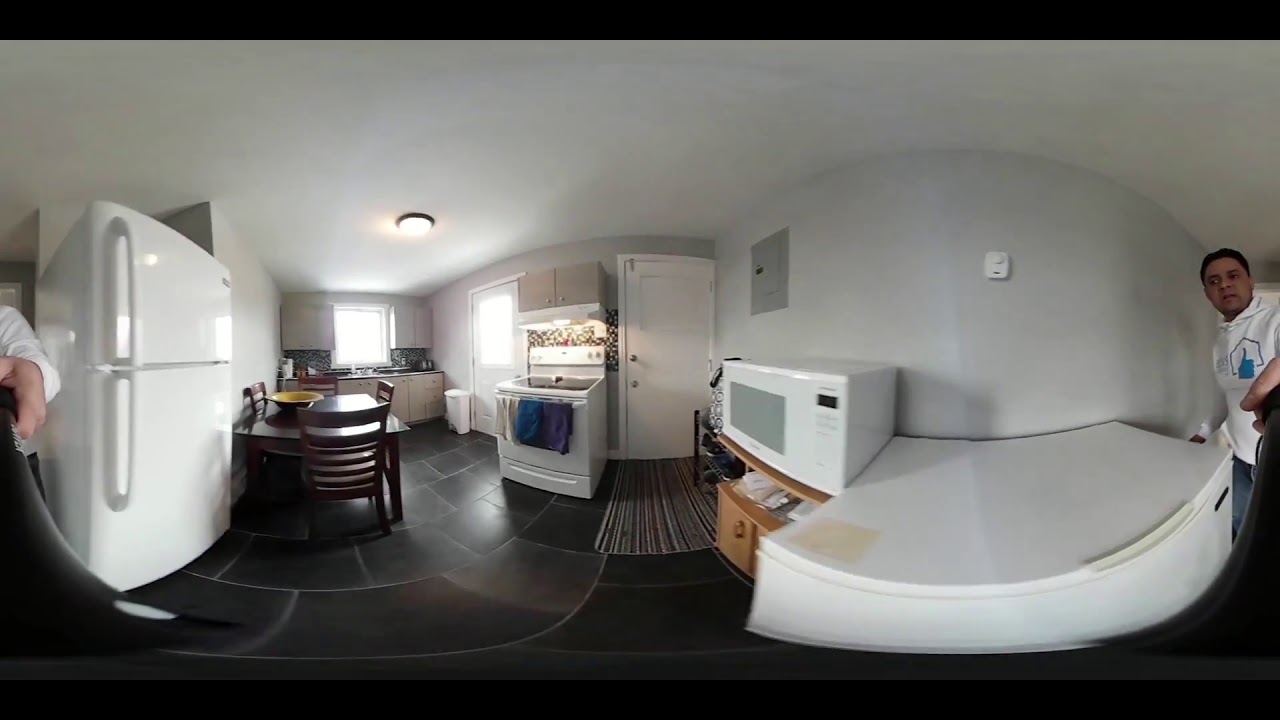A wide-angle photograph captures the interior of a compact apartment with distinctive black tile flooring. The focal point of the image is a man with slicked-back dark hair, wearing a white hoodie featuring a blue thumbs-up graphic, seemingly positioning a stand-up freezer near the center. The apartment's kitchen area is on the right, including a white refrigerator with a top freezer, a small brown dining table set for two with an empty bowl centered on it, and a stove with an oven, which has navy blue and white towels hanging from its handle. The kitchen also features a microwave, a white sink under cupboards, and a coffee maker. A door mat lies in front of an adjacent white door. The apartment has multiple cabinets and two windows that allow natural daylight to illuminate the space. Despite its limited size, the apartment appears well-organized and efficiently furnished. Off to the left, only the arm of an individual in a white shirt is visible. On the far right stands another individual with darker skin and hair, dressed in a white polo shirt, interacting with a white, curved tabletop object. The entire scene is framed with white walls, enhancing the clean and airy atmosphere.